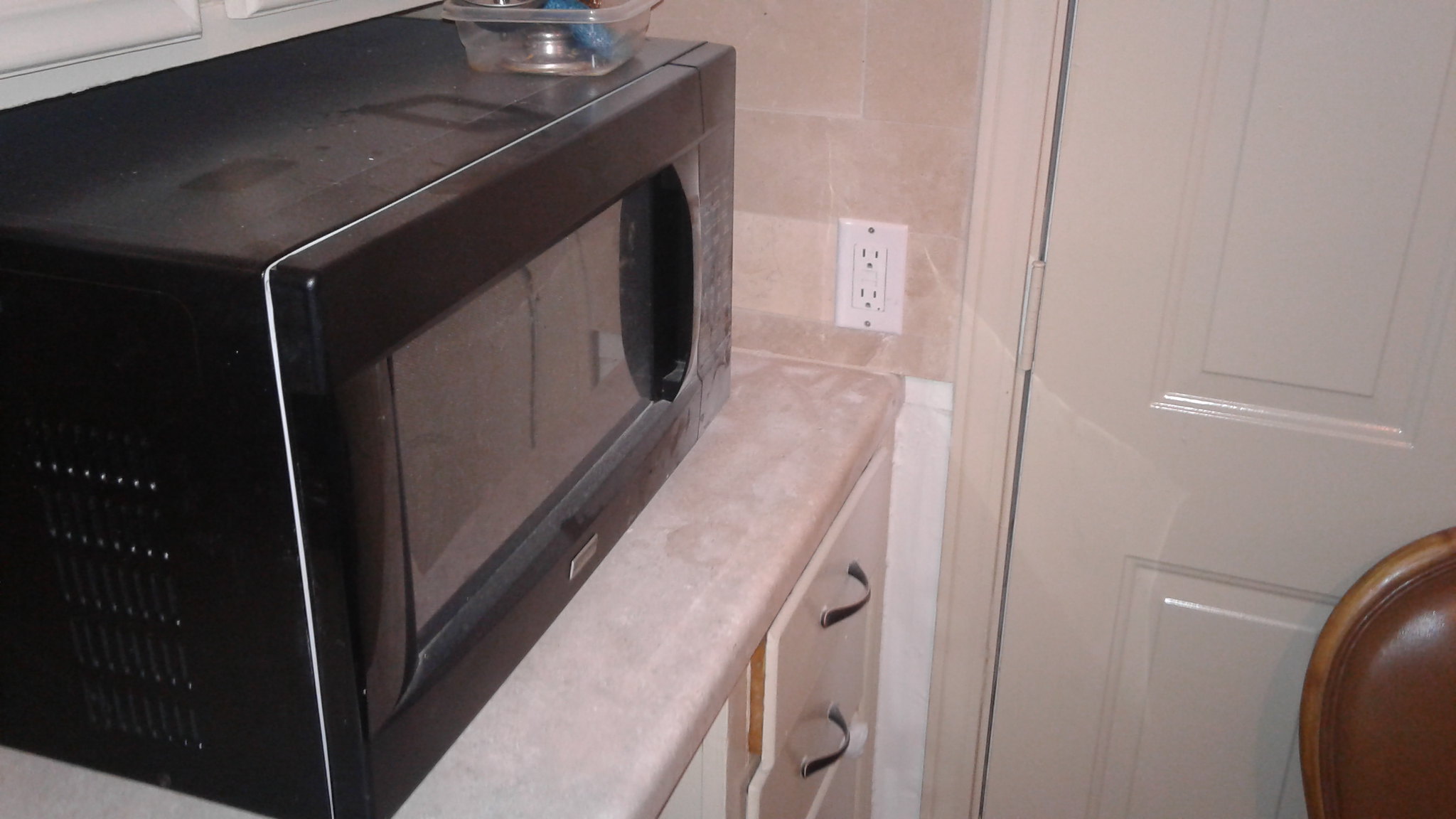This detailed horizontal photograph captures a corner of a kitchen, showcasing a variety of elements dominated by a dusty black microwave. The microwave is positioned on a beige, possibly Formica, countertop and appears to be taken from a left-side, 45-degree angle, emphasizing its side, front, and top. A notable feature on top of the microwave is a plastic container with a few unidentified items inside, including a visible blue object. 

The countertop beneath the microwave is beige or a delicate rose blush color, harmonizing with the kitchen's monochromatic beige theme. The kitchen wall behind the microwave consists of beige tiles in the top left and white paint reaching downward. Just above the counter are additional cabinets rendered in a soft beige color with dark, possibly metal, handles. 

On the wall to the right, there's a vertically oriented electrical outlet with nothing plugged in. A cream-colored door, framed by trim, stands in the background accompanied by the hinge details. Extending further into the photo's periphery, the rounded back and brown cushioning of a wooden chair can be spotted near the door.

Below the microwave, there are several drawers on the cabinet, matching the countertop's beige tone and equipped with dark metal handles. The top drawer is slightly ajar, suggesting use. Additionally, various sources mentioned cabinets above the microwave, likely white, corroborating the kitchen's overall palette.

The scene's subtle clues—a dusty microwave, partially open drawers, and tidy arrangement—paint an intriguing narrative of everyday life paused in mid-motion.